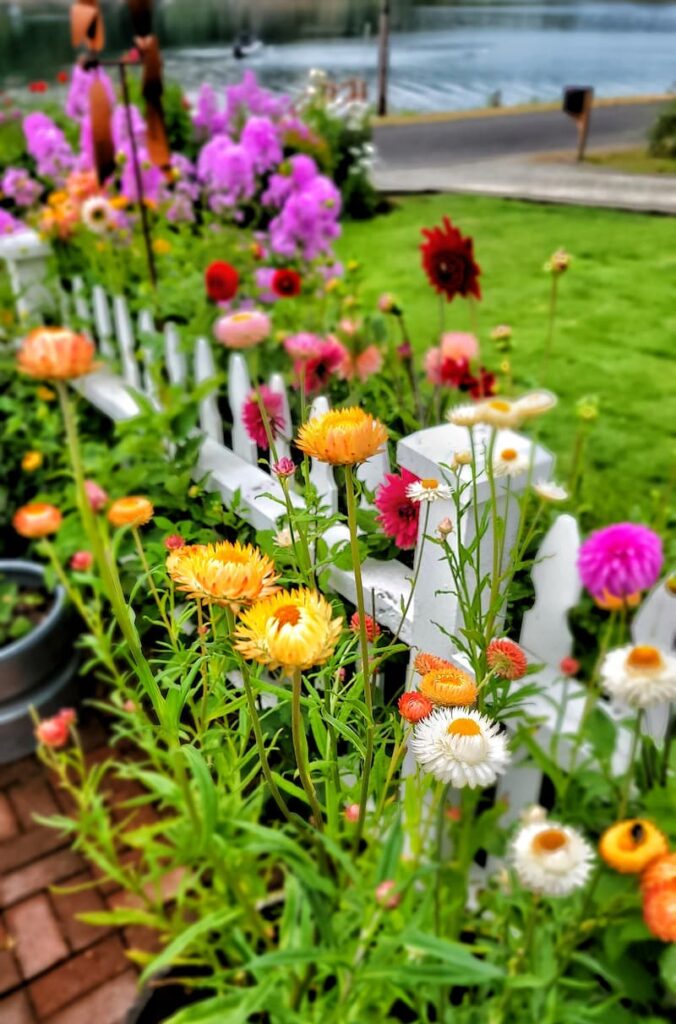The vibrant and colorful garden scene is set on an overcast day, but the photo has been enhanced to look more lively and bright. A white picket fence runs diagonally from the top left to the bottom right, dividing the scene into sections. On one side of the fence, a variety of wildflowers in shades of pink, purple, orange, red, yellow, and white bloom profusely, with some flowers in planters and others in the ground. The fence is bordered by a brick sidewalk, adding a touch of rustic charm to the garden. In the background, a light blue lake dotted with the darker blue streaks can be seen, possibly with ducks on it. To the right, there is a road leading to a driveway with a mailbox, and a swath of lush green grass extends up to the water's edge. The top left corner features a dense dark green that transitions to lighter green grass as it moves inward. The bottom right corner is predominantly green leaves, highlighting the myriad of vibrant flowers that create a stunning, multicolored tapestry against the white fence.